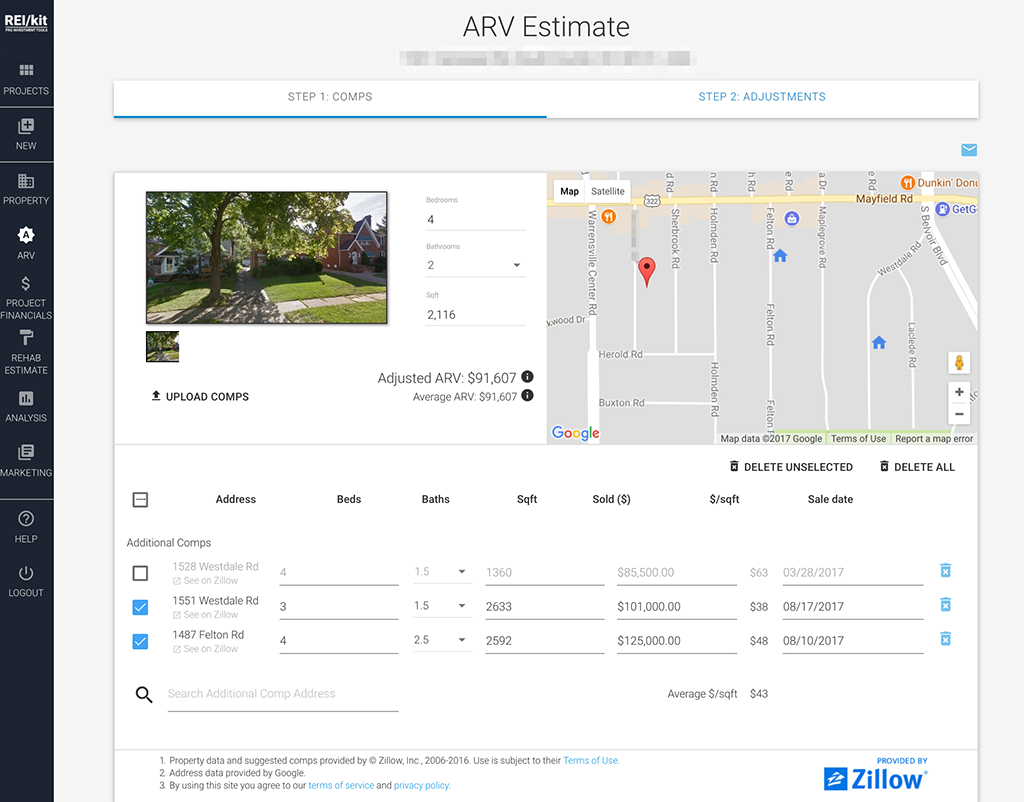**Detailed Caption:**

The provided image is a detailed screenshot from a webpage, likely affiliated with Zillow, displaying the estimated value of a property. In the upper left corner of the page, the header reads "REI/kit." Across the top, bold text in all caps spells out "ARV ESTIMATE," indicating the After Repair Value estimate. Below this header, the webpage outlines a two-step process labeled "Step 1: Comps" and "Step 2: Adjustments."

Prominently featured below the steps is a small photograph showcasing the exterior of a house. The house is framed by large trees in the front yard, with a clear view of the sidewalk and driveway. To the side of the photo, key property details are listed: "Bedrooms: 2, Bathrooms: 2, Square Feet: 2,116." Additionally, the Adjusted ARV (After Repair Value) and the Average ARV are both mentioned as $91,607.

To the right of the property photo is a Google map displaying the surrounding neighborhood. The map includes road labels, with Mayfield Road highlighted prominently running left to right. Points of interest, such as a nearby Dunkin' Donuts, are marked on the map. Other streets like Felton Road, Maple Grove Road, and Sherbrooke Road are also labeled. The map data is credited to Google, with a copyright notice dating to 2017.

Beneath the map, there is a structured table listing various attributes such as "Address, Beds, Baths, Square Feet, Sold, $/Square Foot, Sale Date." Below this table, additional comparable properties (comps) are listed, including their addresses, number of bedrooms and bathrooms, square footage, the sale price, price per square foot, and the date of sale. This comprehensive layout provides a thorough analysis and comparison for estimating the property value.